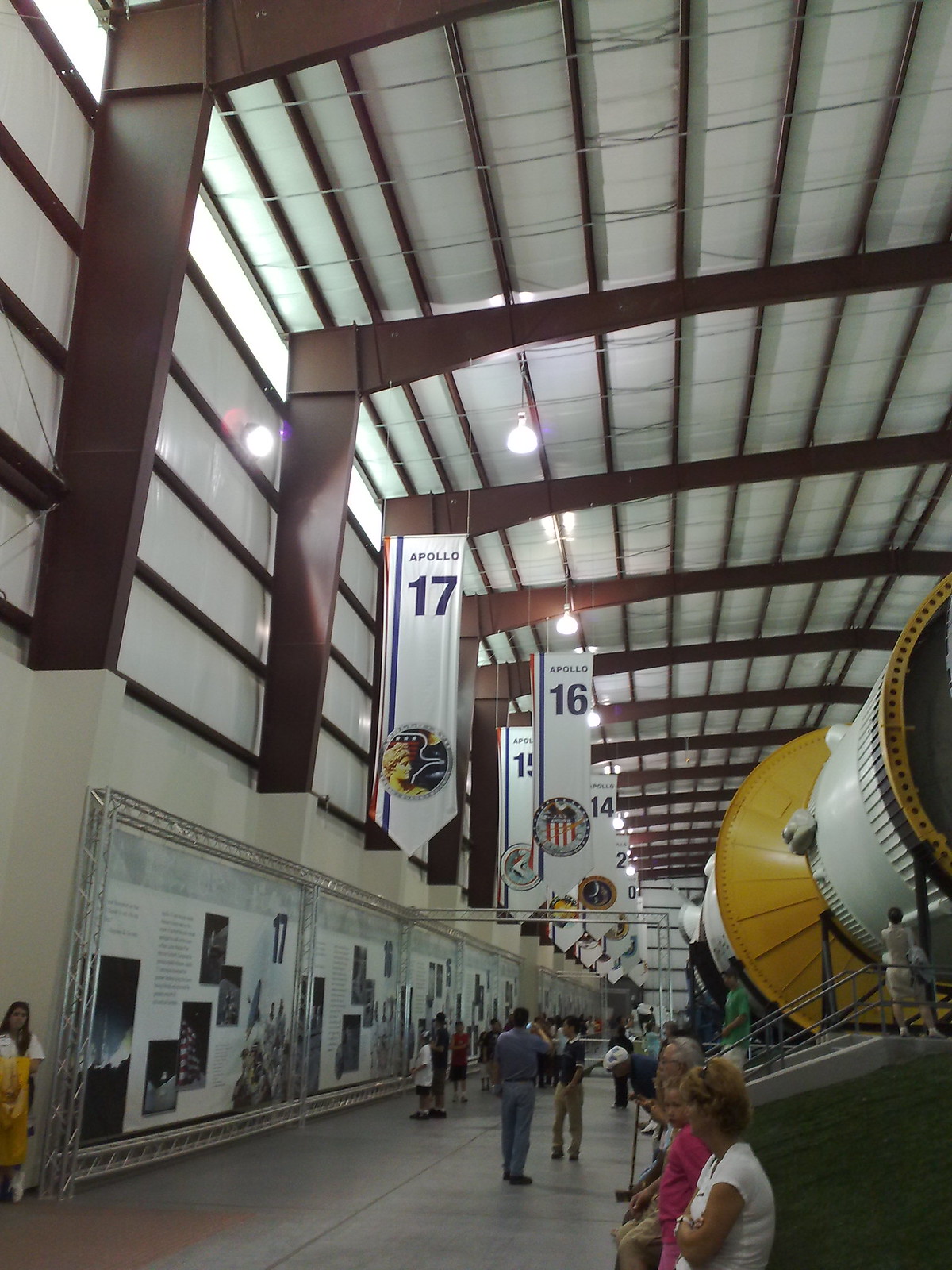The photograph captures the interior of a massive hangar that has been transformed into a museum exhibit showcasing a historic spacecraft. The long, narrow building features white walls and ceilings, interspersed with large brown metal rafters, girders, and connectors. Along the left wall, there is a striking display of text and photographs encased in glass, narrating the story of the Apollo missions. 

Hanging from the ceiling are large pendant banners numbered sequentially from Apollo 17 down to earlier missions, positioned between the supporting beams of the hangar. This organized display of the Apollo mission banners stretches the length of the building, offering a timeline of these historic spaceflights.

On the right side, a prominent large cylindrical structure lies horizontally. This spacecraft component, possibly part of an actual space shuttle or a detailed replica, features a white exterior with a yellow cone section. Visitors are seen both walking and sitting throughout the exhibit, with some people standing on elevated platforms to get a closer look at the rocket, which appears touchable due to its close proximity.

Additionally, informational posters and canvases adorn the walls, filled with images and text that provide context and details about the Apollo missions. The scene is bustling with activity as visitors engage with the exhibition in various ways, contributing to the educational atmosphere of this impressive space.